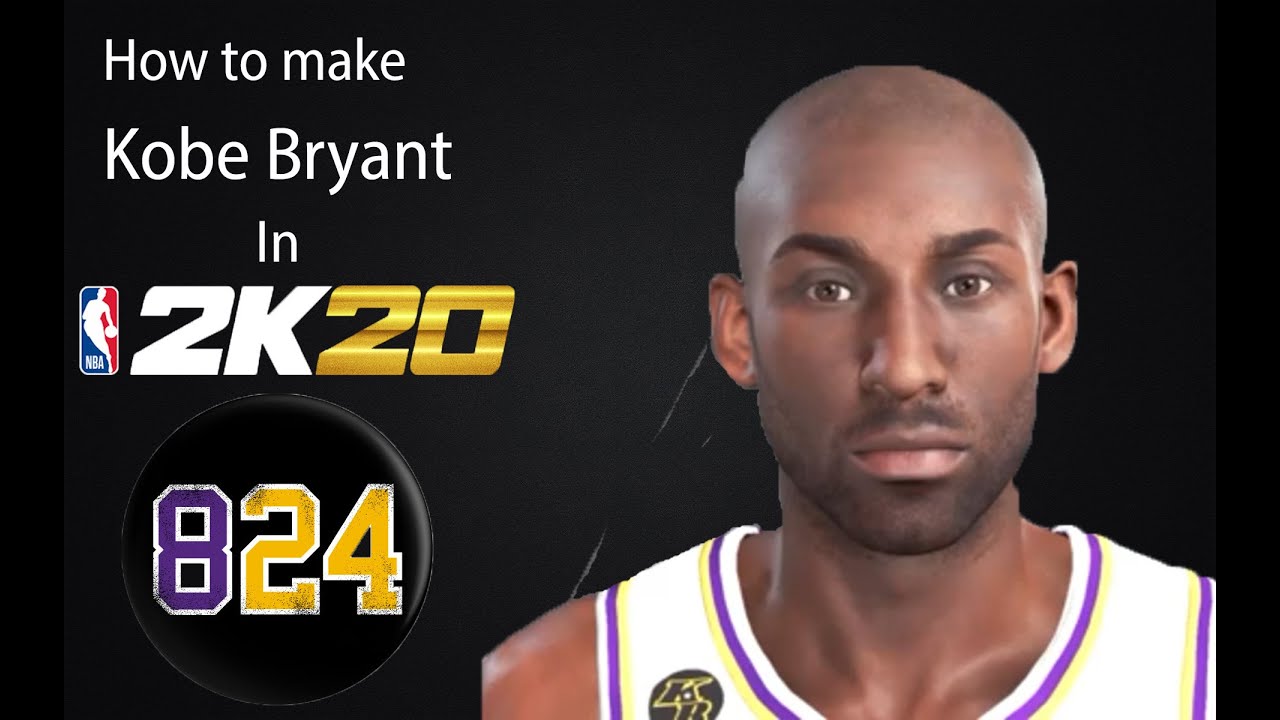The graphic displays a guide on how to recreate Kobe Bryant in NBA 2K20. It prominently features the numbers 8 and 24, representing Kobe's iconic jersey numbers during his career with the Los Angeles Lakers. On the right side of the graphic, there is an in-game character model meant to resemble Kobe, donned in a white Lakers jersey. While the facial features capture a general likeness, certain structural details are slightly off. The character is completely bald, suggesting an older version of Kobe. The purpose of the graphic seems to be to provide instructions for gamers on crafting a fairly accurate rendition of Kobe Bryant. This game was released prior to Kobe's tragic death, so it is unclear if this graphic is intended as a tribute to him or simply a coincidence, unrelated to his passing.